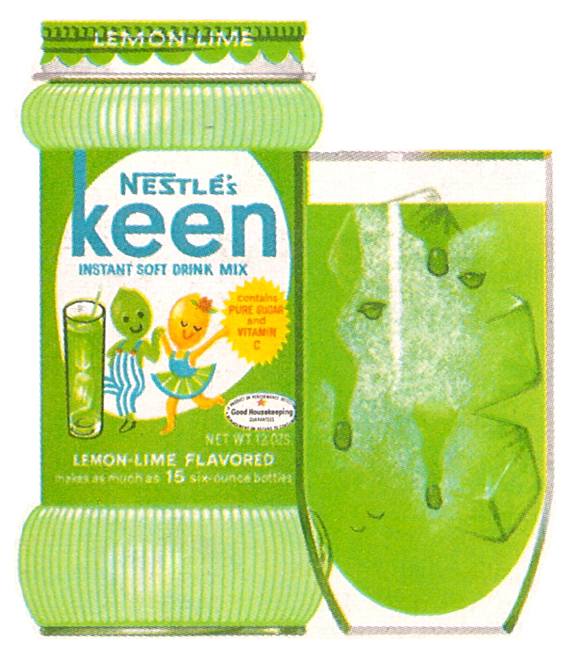The image depicted is a zoomed-in view of an old advertisement, likely from the mid-20th century. On the right-hand side of the image, there is a clear glass filled with a green liquid and approximately three ice cubes. Adjacent to the glass is a jar with a green and silver lid, bearing the label "Lemon with a Dash of Lime."

The jar appears green, though it's uncertain if this is due to the jar itself or the substance inside it. Surrounding the jar is predominantly green packaging, featuring a white oval inscribed with the text "Nestle's Keen Instant Soft Drink Mix" in blue lettering. 

To the left of the jar, there's a cup that also contains the green liquid. Next to the cup stands a whimsical green character with a black smiley face, and black and white eyes. This character is dressed in a blue and white striped jumper with red buttons.

Beside this character is a personified lemon and lime. The lemon is illustrated with a cheerful demeanor, while the lime character wears a rose atop her head and dons a dress colored in blue, green, and white hues. The entire scene conveys a playful, vibrant ambiance typical of vintage advertisements.